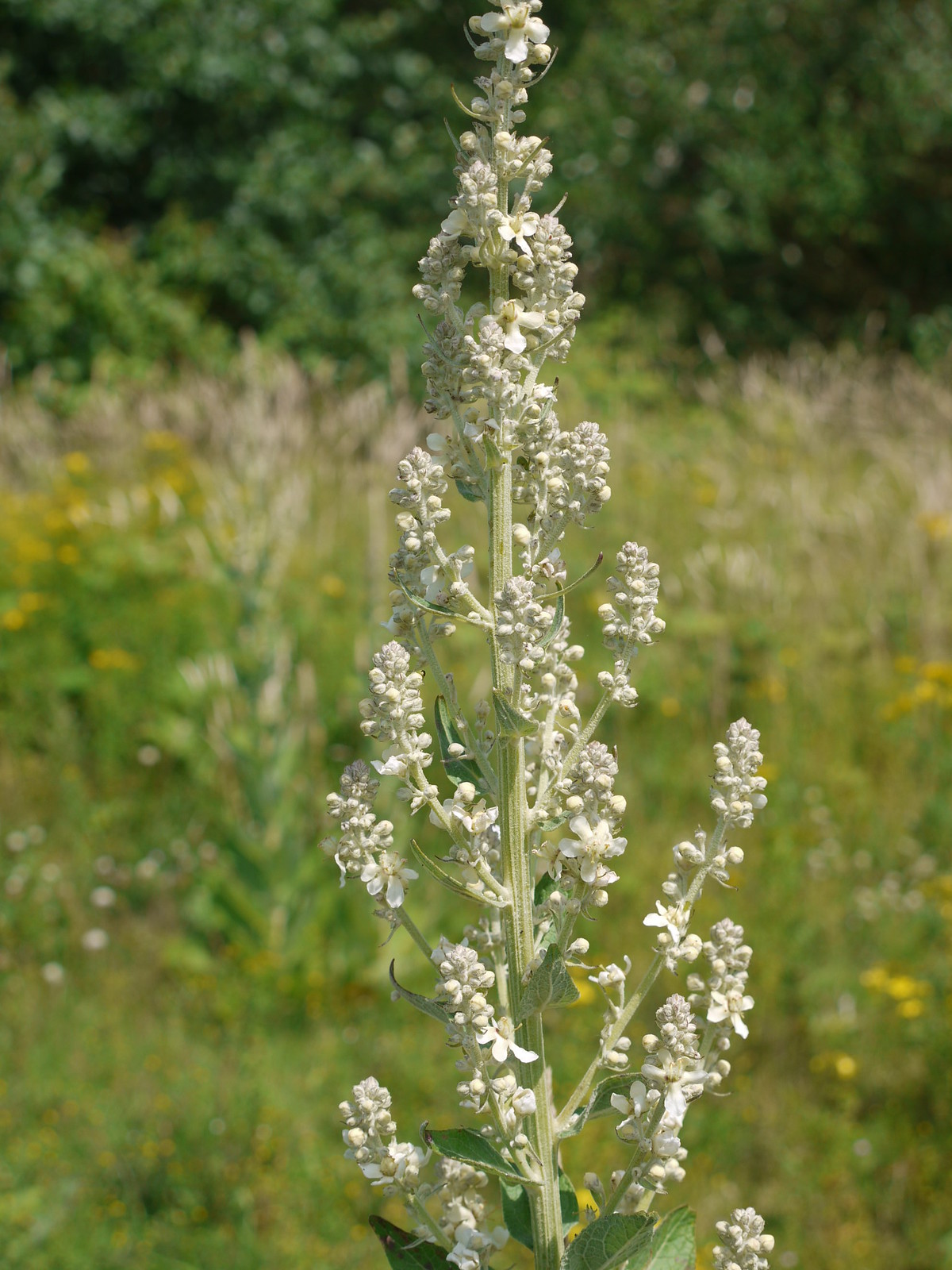In the foreground of this outdoor scene, a tall, roughly three-foot plant stands as the central focus, its sturdy, light green stem extending straight upward. The plant features an array of small, white flowers and buds that form delicate clusters along its stalks, accompanied by a few dark green leaves towards the base and middle. The sunlight highlights the plant, making its intricate details and vibrant colors stand out clearly. Surrounding the plant is a field of high grasses and weeds, interspersed with sporadic yellow wildflowers, possibly dandelions, adding patches of color. The background, while blurred, reveals deeper green foliage and occasional dark patches, suggesting distant trees that frame the wild and untamed landscape.